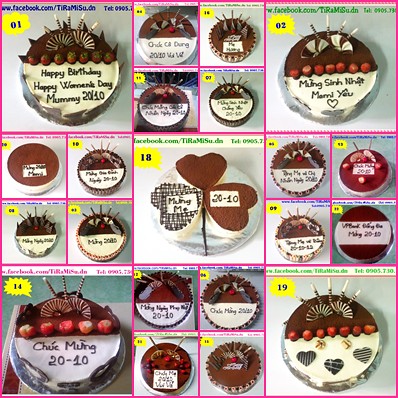The image is a detailed and intricate poster displaying approximately 19 different cake designs arranged in a square layout, subdivided into smaller squares. The arrangement follows a pattern where some squares are further divided into four smaller squares. The cakes predominantly feature a color palette of dark plum, brown (chocolate), and white. Many cakes have white frosting on the bottom with chocolate decorations on top and include strawberries or raspberries. Specific designs include a cake inscribed with "Happy Birthday, Happy Women's Day, Mommy 2010", showcasing a blend of white frosting and dark chocolate, adorned with strawberries. Another notable design involves a pattern where three heart-shaped cakes, one frosted white with accents of white and brown, and two in brown, come together to form a shamrock shape. The poster also mentions a website and a telephone number, providing a contact source for more information. The cakes are intricately decorated with varying designs and messages, and each section of the poster highlights the attention to detail and aesthetic appeal of the confectionery creations.